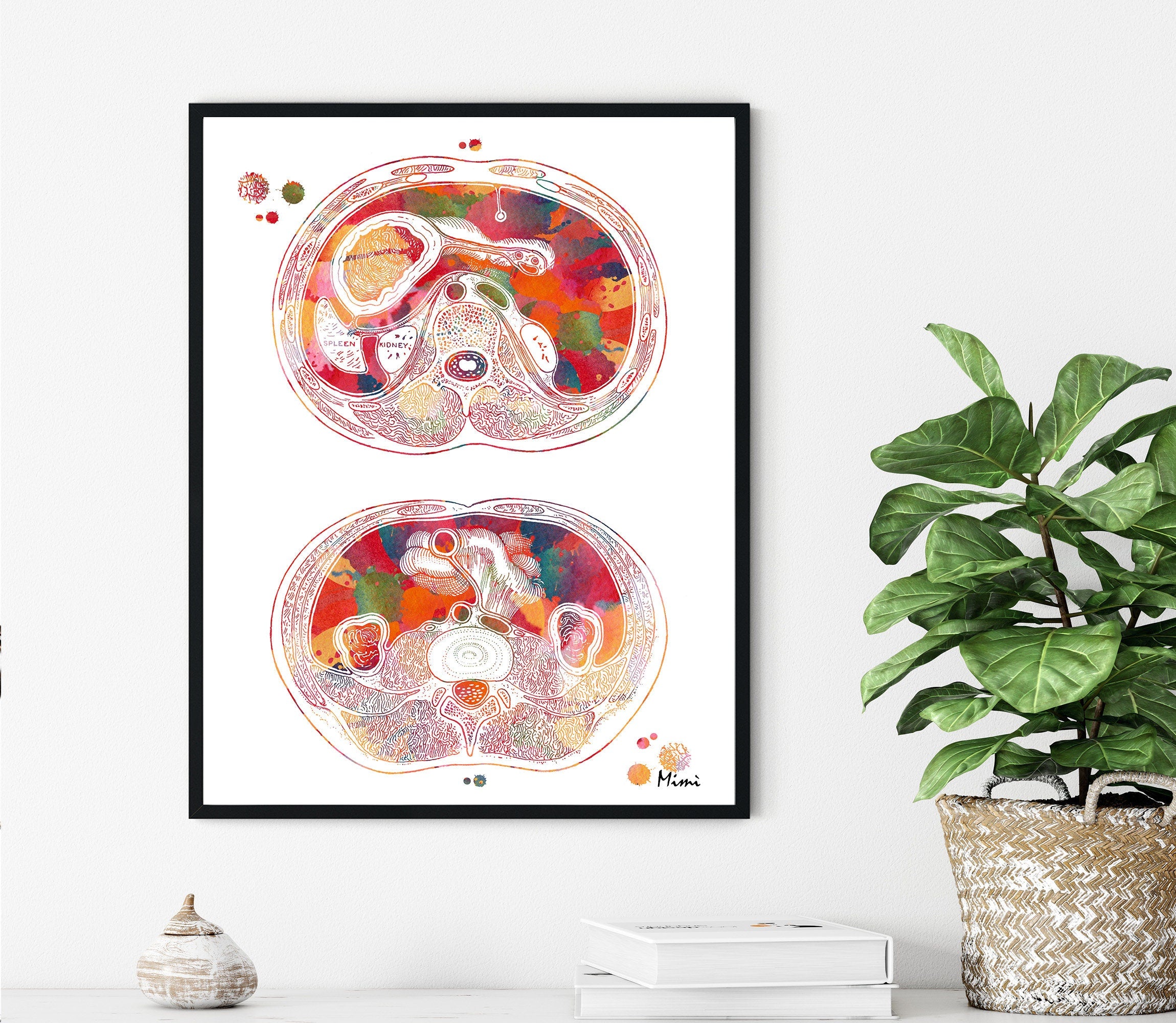Against a light gray or white wall, there is a striking black-framed painting that serves as the focal point of the image. This painting is done on white paper and displays two abstract, circular shapes that resemble cross-sections of a human brain. These shapes are filled with vibrant colors including red, green, orange, purple, and blue concentrated in the center, with more muted, lighter tones around the edges. The composition exudes a sense of complexity and detail similar to microscopic slides or CAT scan images.

In the lower right corner of the painting, the signature "Mimi" is inscribed in black ink. To the painting's left, a series of colorful dots appear: a red spot, a green dot with a red top, two red dots of varying sizes, and a dot that is half red and half yellow. Below these, there is a green dot enclosing a yellow dot, and another small green dot. On the right side of the painting, there are orange and yellowish dots, with one featuring red and yellow spots.

Below the painting, a white tabletop holds a variety of items. On the left side, there is a small pot, its details not entirely clear, accompanied by a stack of two white books. On the right side, a wicca basket houses a green, leafy plant, adding a natural touch to the setting.